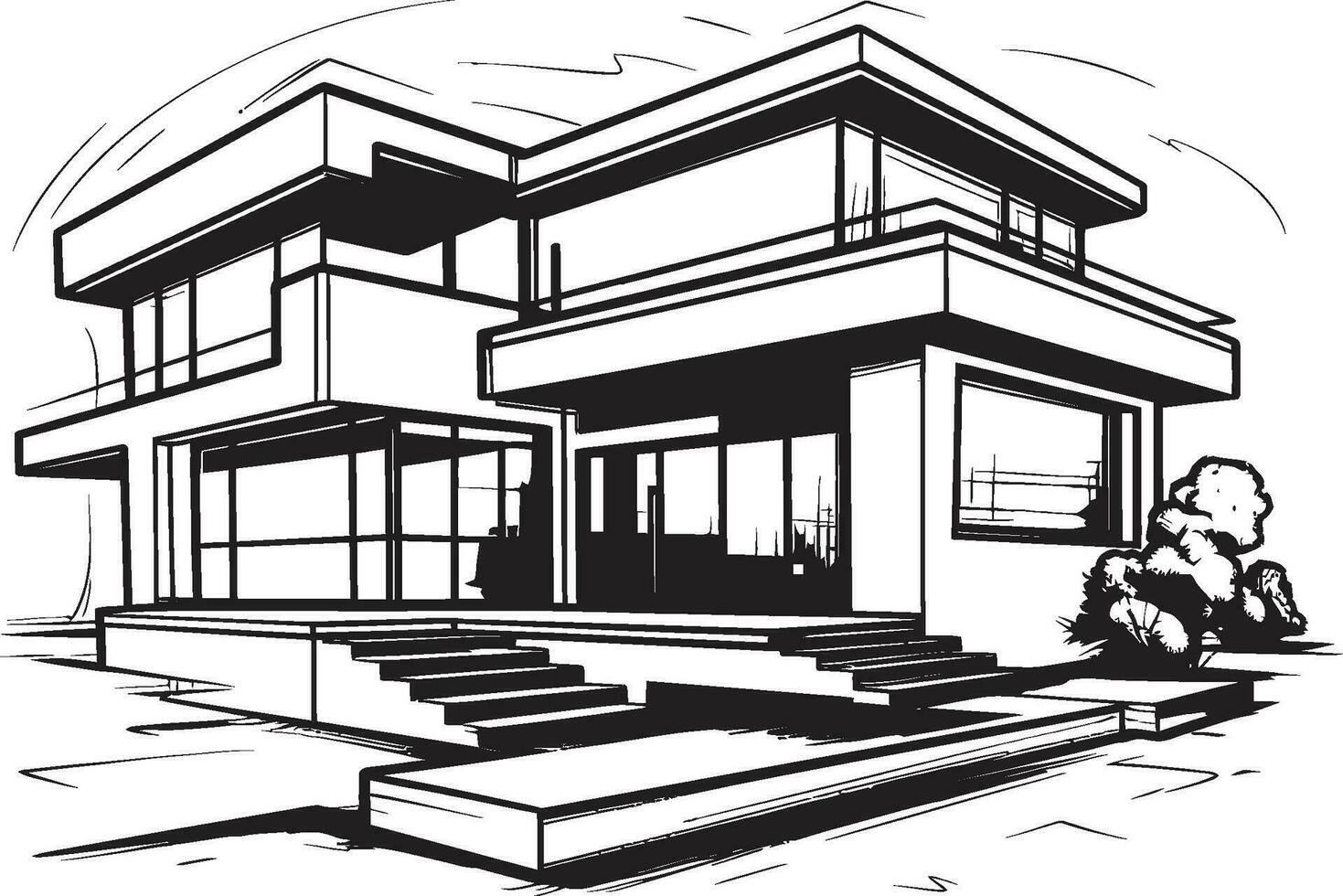The image is a detailed black-and-white sketch, likely an architect's drawing, of a very modern, geometrically styled two-story house. The house features an abundance of large, floor-to-ceiling glass windows that wrap around most of its perimeter, creating an open and airy feel. It has a flat, square roof and is designed with clean, angular lines, emphasizing a contemporary aesthetic. Two stairways lead up to the first level, converging on a platform that serves as an entryway. The second level boasts a wraparound balcony with a railing, enhancing the modern design. There are a few shrubs and small plants strategically placed in front of the house, particularly on the right side of the image. The structure appears almost entirely composed of square and rectangular shapes, with minimal solid walls, highlighting the extensive use of glass and modern architectural elements.